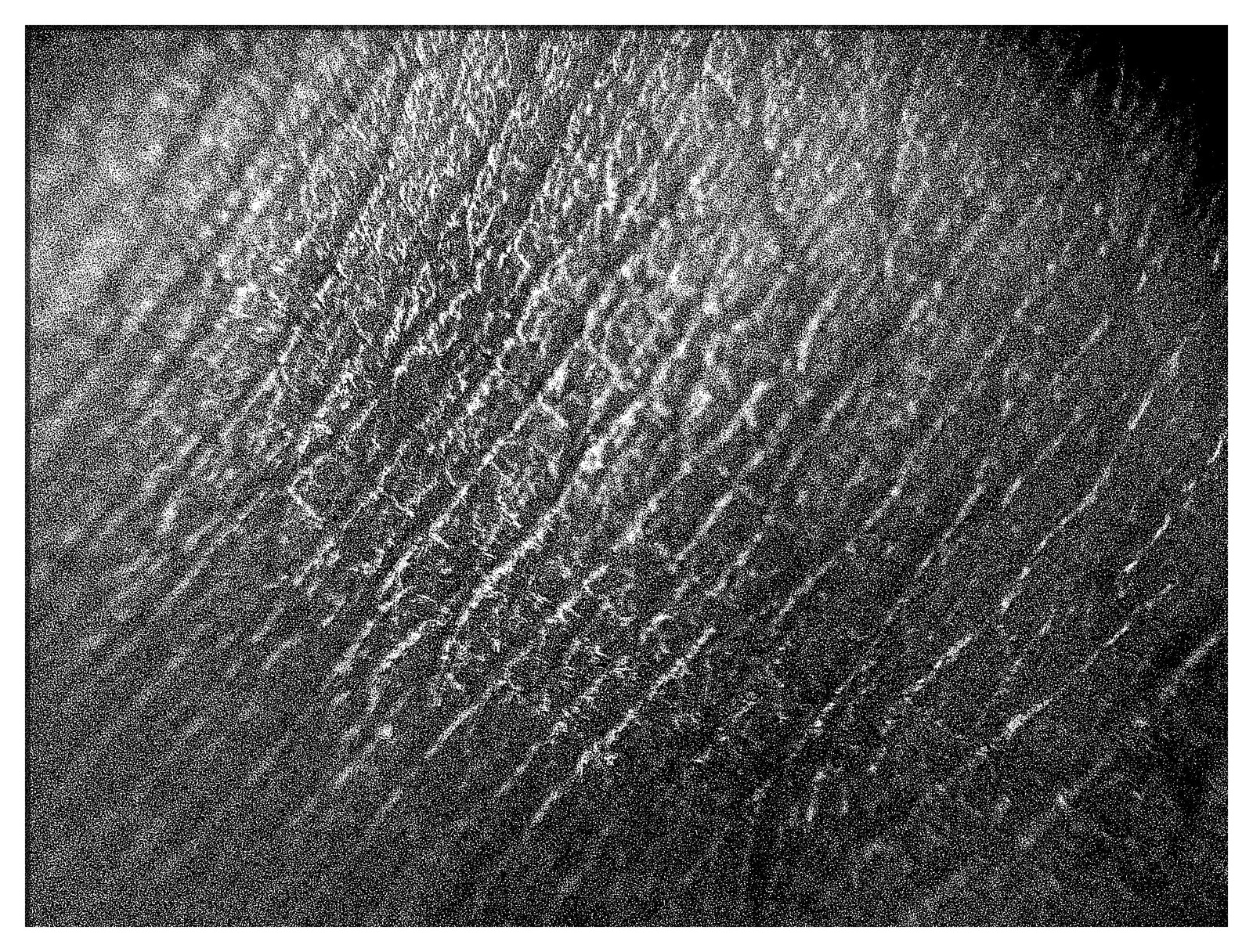The black-and-white photograph presents an extreme close-up view of skin, emphasizing the intricate patterns and textures. The image is dominated by fine wrinkles that traverse diagonally from the bottom left to the center and up to the top right. The skin's surface appears with a grayish tone interspersed with highlighted white creases, illuminated by a light source centered on the image. The background fades into deep black particularly in the top right, bottom right, and top left corners, creating a stark contrast with the detailed skin texture. The photograph's tight focus on the wrinkled surface provides no context about the subject’s identity, making it impossible to discern whether the skin belongs to a human or an animal, let alone details such as age, race, or gender.